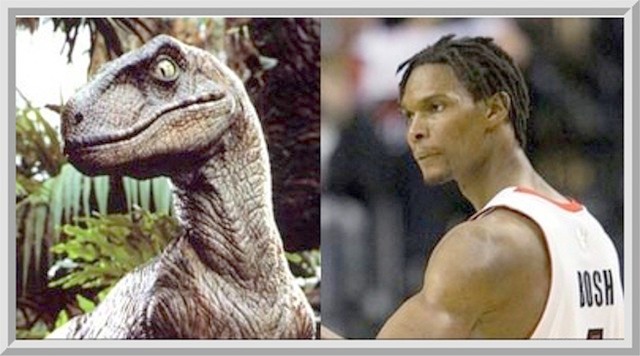The side-by-side image comparison features a dinosaur and NBA player Chris Bosh. On the left, there is a dinosaur with a somewhat elongated neck, which could be described as a stretched-out neck, looking to the side in a three-quarter view pose. On the right, Chris Bosh, an African-American basketball player, is similarly posed in a three-quarter view, also looking to the side. He is wearing his white basketball jersey, with his name "Bosh" visible on the back. His shoulder and bicep muscles are prominently displayed, emphasizing his athletic build. The background of the image featuring Bosh is blurred, offering no discernible details. The comparison seems to draw a visual parallel between the dinosaur's neck and Bosh's long neck.